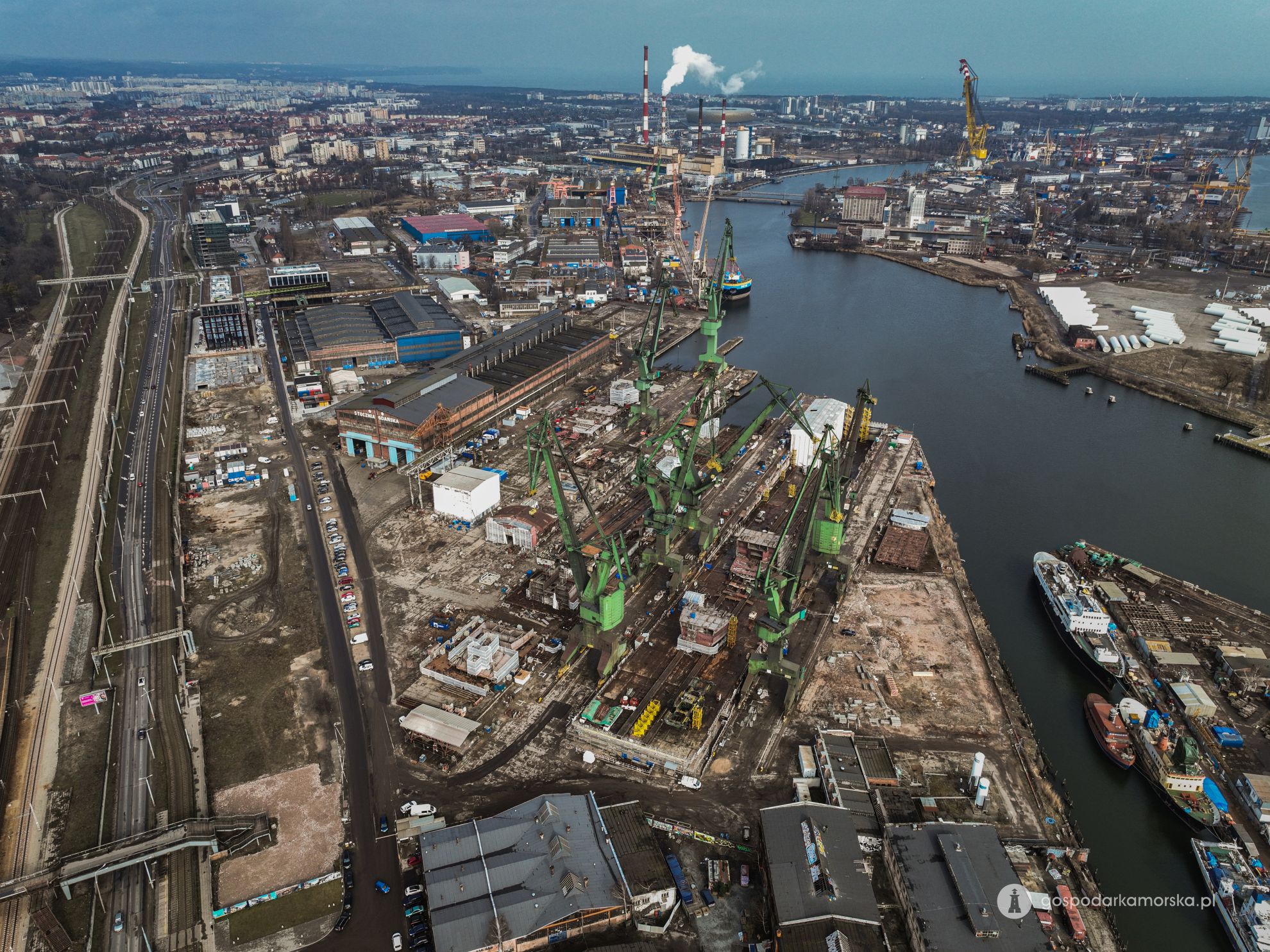The image is a detailed, bird's eye view of an industrial shipyard and port area, bustling with activity. Positioned centrally are numerous cranes, surrounded by a variety of buildings and structures. To the bottom left, a road extends upward, seemingly leading toward a distant city center situated in the top left corner. To the right of the cranes, starting from the middle and continuing down, there's a canal filled with docked ships, lined with barrels on the dock. On the opposite side of the canal, in the top right, are more industrial buildings and cranes. A prominent red and white smokestack emits white smoke, centrally visible at the top of the image. The color palette includes shades of green, yellow, gray, blue, brown, red, and black, giving the entire scene a slightly aged, possibly 1980s or '90s, and gritty industrial atmosphere. The sky is a dull blue, adding to the overall somber mood of the photograph. The image also features various roads, highways, and parked cars, with the water stretching out in the distance, reinforcing the shipyard's connection to the ocean.